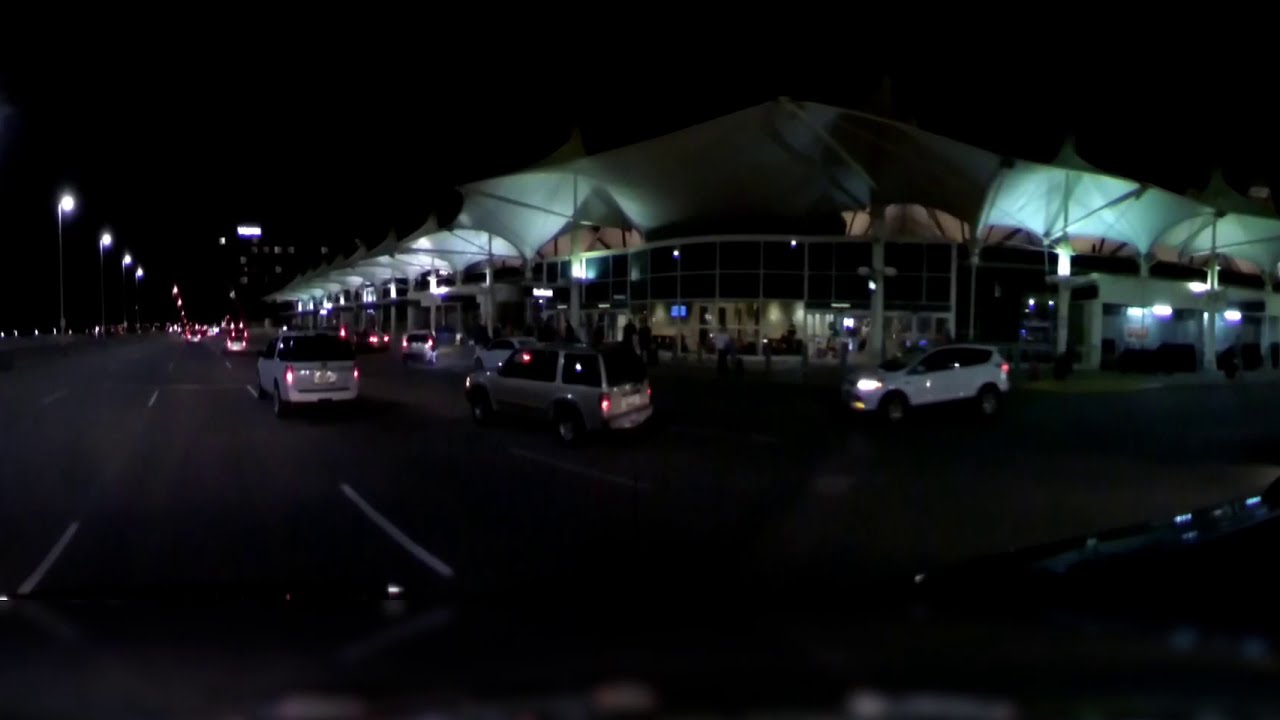The nighttime image depicts a view from inside a vehicle, focusing on a bustling three-lane road in front of an airport. The bottom portion of the image reveals the dark hood of the car. Stretching across the right side of the image, the airport building is adorned with numerous white, triangular-shaped canopies. The structure extends down an intersecting street, and its facade features many glass windows and doors, with a rounded corner from which interior lights and figures are visible. The road in the foreground is alive with traffic, consisting of various vehicles traveling from the right side towards the back left, illuminated by numerous street lamps lining the left side of the road. The upper portion of the image is shrouded in the darkness of the night sky.